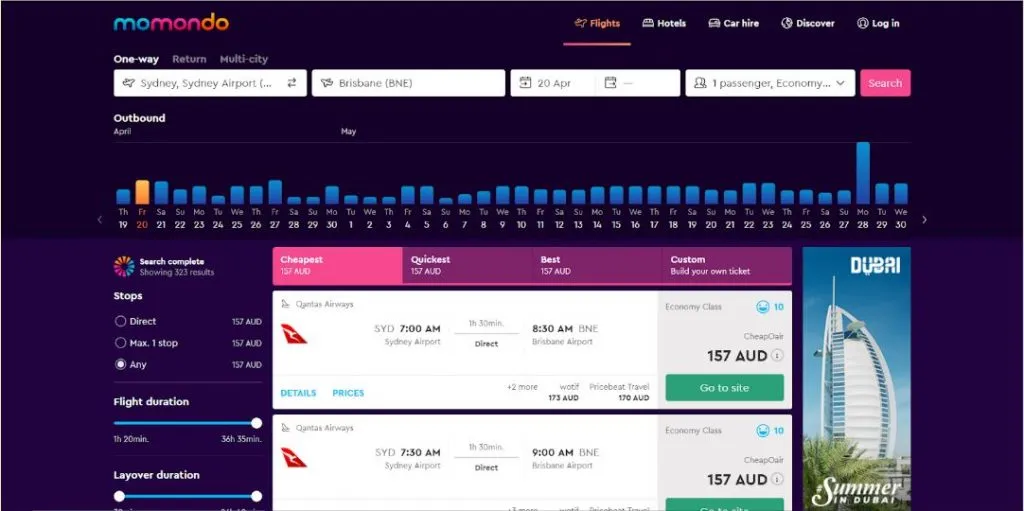The image appears to be a screen capture of a flight search results page, with a distinctively styled interface dominated by shades of purple and pink. 

At the very top, the header showcases the name "Mondo," written in vibrant gradients of blue, pink, and orange hues. Below the header, a pink navigation bar lists various sections: "Flights" which features a small flight icon, "Hotels" with a bed icon, "Car Hire" with a car icon, "Discover" with a globe icon, and "Log In" with a person icon, all in white text.

Beneath the navigation bar, there are several user input fields and options. Users can select between "One Way," "Return," and "Multi-City" trip options, indicated in white text. Following this, four input fields are presented with placeholder text in gray:
1. "Sydney, Sydney Airport," accompanied by an airplane icon.
2. "Brisbane, BNE," also with an airplane icon.
3. "20th APR," flanked by calendar icons.
4. "One Passenger, Economy," with a person icon.

A prominent pink and white search button invites users to commence their search.

Further down, information regarding outbound flights is displayed alongside a graph in orange and blue, representing flight availability over April and May. Below the graph, the text reads "Search Complete," indicating 323 results found.

Filters are available for refining the search, inclusive of stops (with "Direct," "Max 1 Stop," or "Any" as options, the latter of which is checked). There's also a price filter, displaying "157 AUD," and a slider for flight delay duration, adjustable between 1 hour 20 minutes and 36 hours 35 minutes. Layover durations can also be configured, though the exact numbers are partially obscured.

Towards the bottom of the interface, there are four primary sorting options highlighted in pink and purple bars: "Cheapest" (in white), "Quickest," "Best," and "Custom," all styled in white text on purple backgrounds.

The search results are presented on white backgrounds, starting with a red and white airline logo. The details for each flight include departure from SYD at 7 a.m., direct flight status, arrival at BNE at 8:30 a.m., and the cost of 157 AUD. A green box labeled "Go to site" offers users the chance to proceed with booking. Subsequent entries provide similar flight options, such as another flight from Sydney at 7:30 a.m., arriving in Brisbane at 9 a.m., also priced at 157 AUD.

The image encapsulates a fairly comprehensive and user-friendly flight booking interface, emphasizing ease of navigation and a plethora of customizable options for potential travelers.